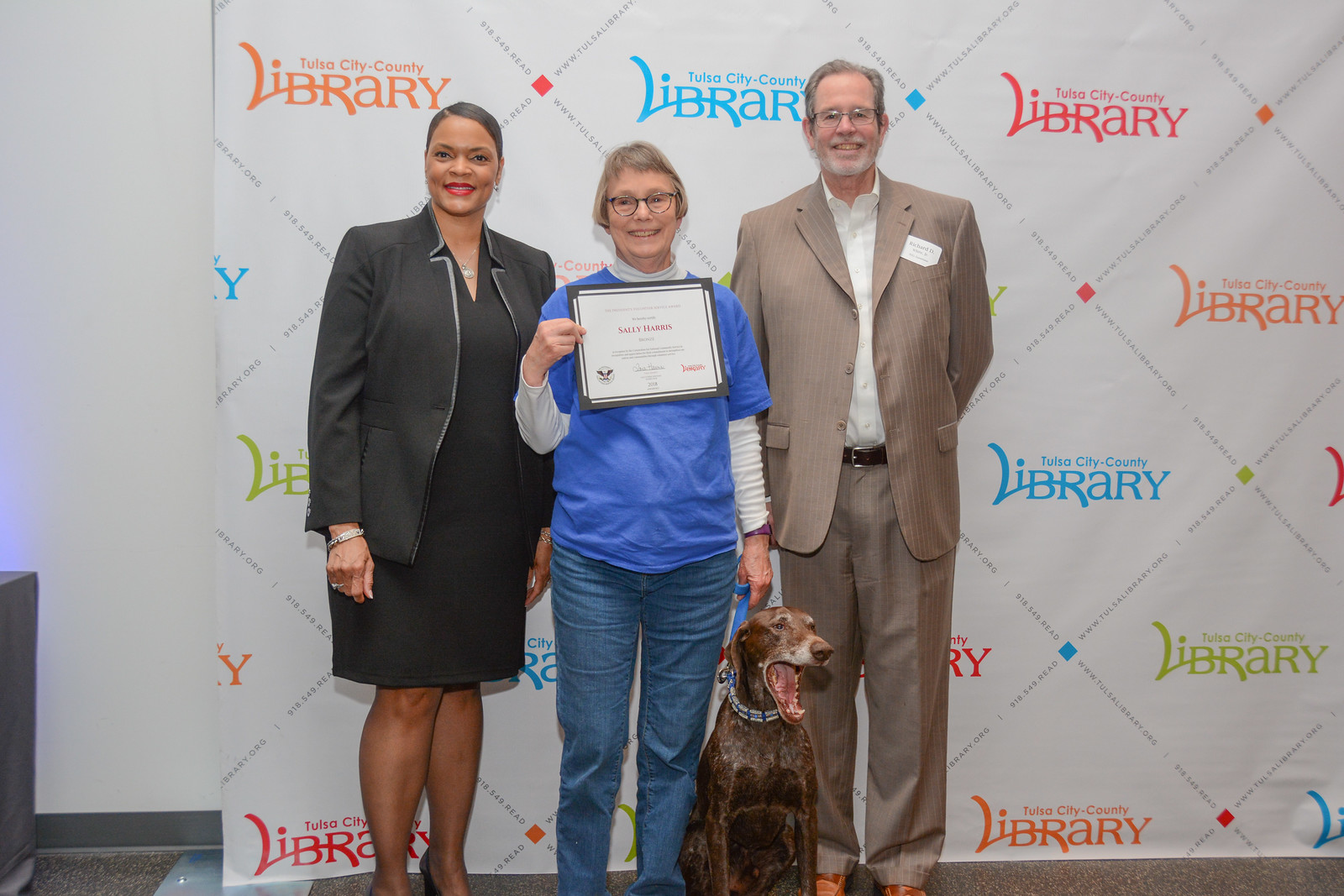In this image, an award ceremony is taking place on a stage with three people standing together in front of a press banner adorned with the multicolored text "Tulsa City County Library" in green, blue, red, and orange. The scene is complemented by a white wall with a gray Cove Base at the bottom.

On the right stands an older man in a brown suit accompanied by brown shoes. He has a white button-up shirt, no tie, graying hair, glasses, and a gray beard.

At the center, an older woman named Sally Harris is holding a certificate, featuring her name in red writing. She wears a blue t-shirt over a white long-sleeve shirt paired with blue jeans. She sports short hair, streaked with gray and brown, and glasses, and she is smiling warmly. Additionally, she holds the leash of a brown dog with white around its nose.

On the left, an African American woman, likely in her late thirties, features short black hair tied back. She is dressed in a black skirt or dress and a black suit jacket, contributing to the formal atmosphere of the event.